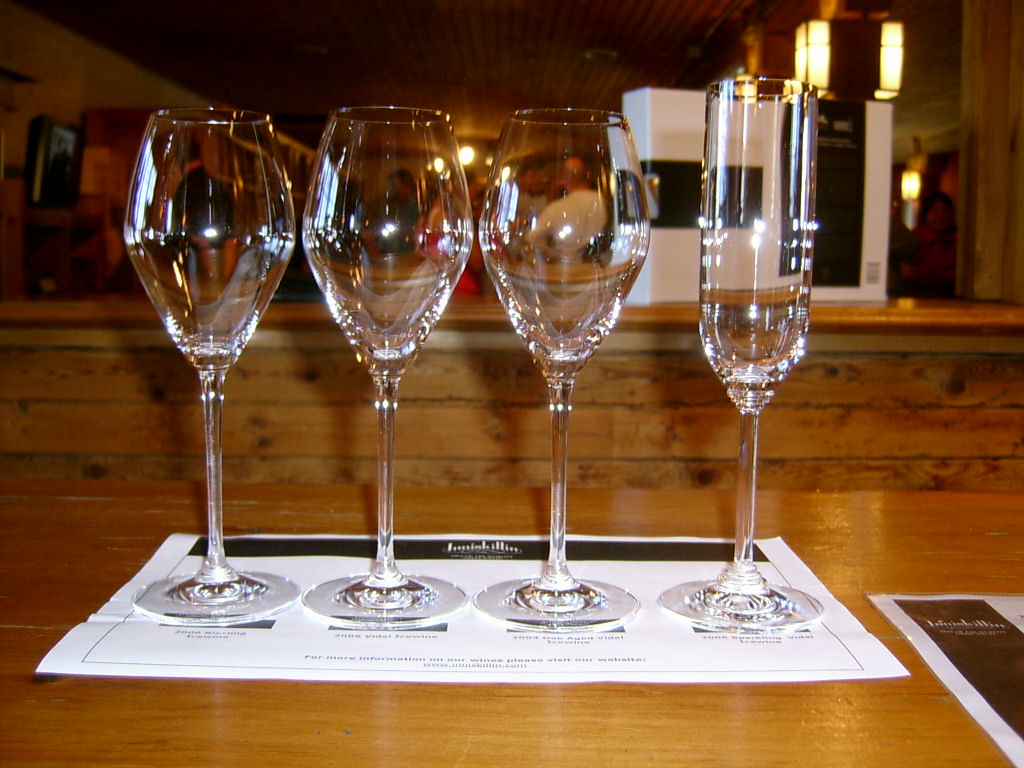The image shows four distinct wine glasses arranged in a row on a wooden surface, likely a bar or restaurant table. The three on the left are wide-bowled wine glasses with long, slender stems, while the one on the far right is a taller, narrower flute glass. They are placed on a white sheet of paper with some indiscernible black text, possibly a menu or a label indicating the type of beverages they might contain. Behind the glasses, there's a white and black box and a television set mounted on the wall to the left. The background reveals a blurred scene of a restaurant with patrons; one discernible figure, seen through the glasses, is a balding man in a white shirt with his back turned. The environment appears warmly lit, featuring wooden elements that extend to the walls and ceiling, and some hanging square-shaped lights contribute to the cozy ambiance.